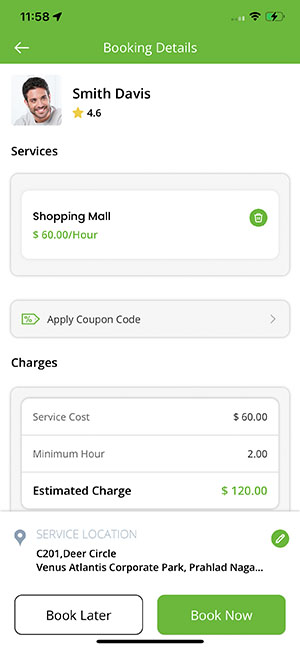The image displays the booking details for services at a shopping mall. At the top, there is a green banner with an icon resembling a power button on an electronic device. The display indicates full internet connectivity and shows the current time as 11:58. Below this section, the booking details are prominently featured.

The service provider is "Smith Davis," who has a 4.6-star rating. The service offered is specifically related to shopping malls, priced at $60 per hour. These details are enclosed within a white box bordered in gray.

Directly underneath, there is a gray box encouraging users to "Apply Coupon Code," accompanied by a green tag icon with a percentage symbol on the left and a right arrow indicating navigation.

The charges section is segmented into three parts within a white box bordered in gray. The service cost is listed in gray at $60 per hour, with a minimum booking of 2 hours. The "Estimated Charge" amounts to $120 and is highlighted in green, while the label "Estimated Charge" is in black.

Further down, the service location is detailed as "C201 / Deer Circle, Venus Atlantis Corporate Park, Prahla, Naga," followed by ellipses indicating continuation. At the bottom, there are two booking options: "Book Later," which is styled with a white background, black text, and a black outline, and "Book Now," which is highlighted in green.